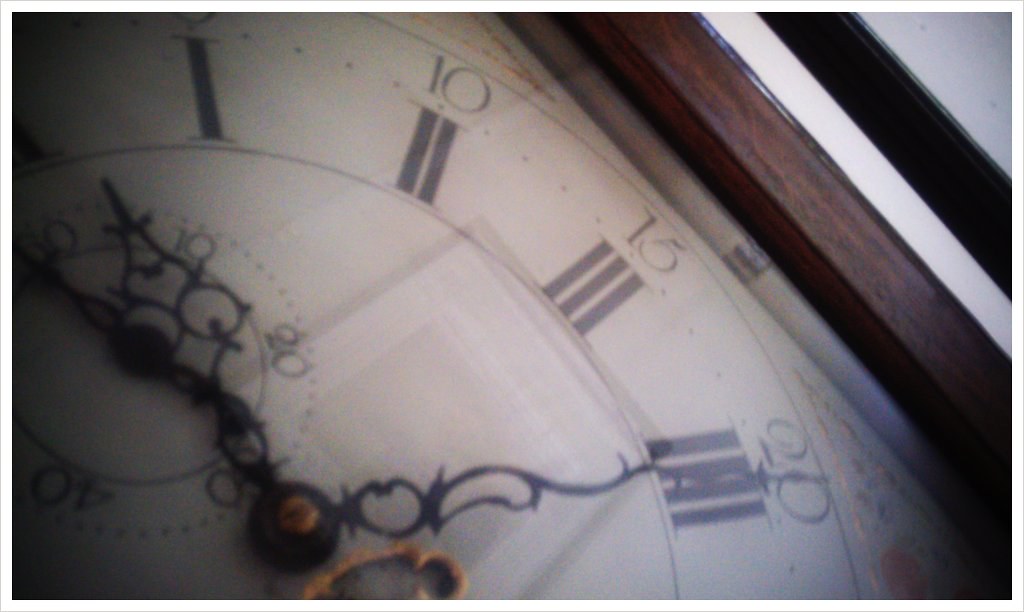This exceedingly wide horizontal image, which is twice as wide as it is tall, exquisitely captures a close-up of a vintage clock face. The clock is encased in a dark brown wooden frame, showcasing its rustic charm. Evident signs of aging are visible on the white face of the clock, imparting a sense of history and timelessness. The face is adorned with Roman numerals in black, complemented by smaller Arabic numerals positioned above each Roman numeral. For instance, the Roman numeral II has "10" written above it, III has "15," and IV bears the numeral "20." 

The clock's hands are exceptionally ornate, featuring intricate patterns of circles and vase-like tips, adding to the antique aesthetic. Only the hour and minute hands are present, and they indicate the time as twenty minutes past twelve. The photograph's composition emphasizes the right side of the clock face, while the left side and lower left corner of the image are shrouded in darkness, creating a dramatic interplay of light and shadow.